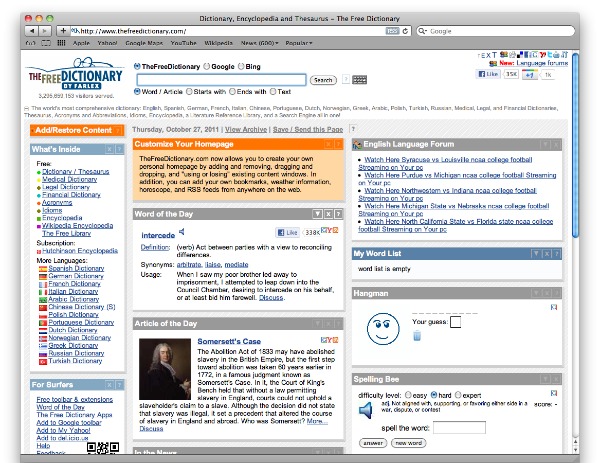A screenshot displays an open webpage on a MacBook operating macOS, identifiable by the distinctive three-button UI in the top left corner (red, yellow, green) and a silvery menu bar with characteristic macOS font. The webpage being viewed is thefreedictionary.com, a comprehensive resource offering dictionary, encyclopedia, and thesaurus functions. 

At the top of this landing page is a search bar, allowing users to select between Google or Bing and refine their search by article, starting or ending words, or full text. Despite somewhat poor resolution, several details are discernible:

- The left-hand column hosts a plethora of links categorized under various dictionaries and encyclopedias, including legal, financial, and Wikipedia resources. Additionally, users can select language options such as Spanish, French, Italian, and Chinese.
- The central column invites users to personalize their homepage. Prominently featured here is the "Word of the Day," which today is "intercede," defined as "act between parties with a view to reconciling differences." Further down this column, there's a historical reference to "Somerset's case" pertaining to the Abolition Act of 1833, which culminated in the cessation of slavery within the British Empire.
- On the right side, the third column kicks off with the "English Language Forum," featuring various discussion threads. This section also includes interactive features like "My Word List," "Hangman," and a "Spelling Bee" game, available in easy, hard, or expert levels. Users have the option to hear a word pronounced and then type it correctly.